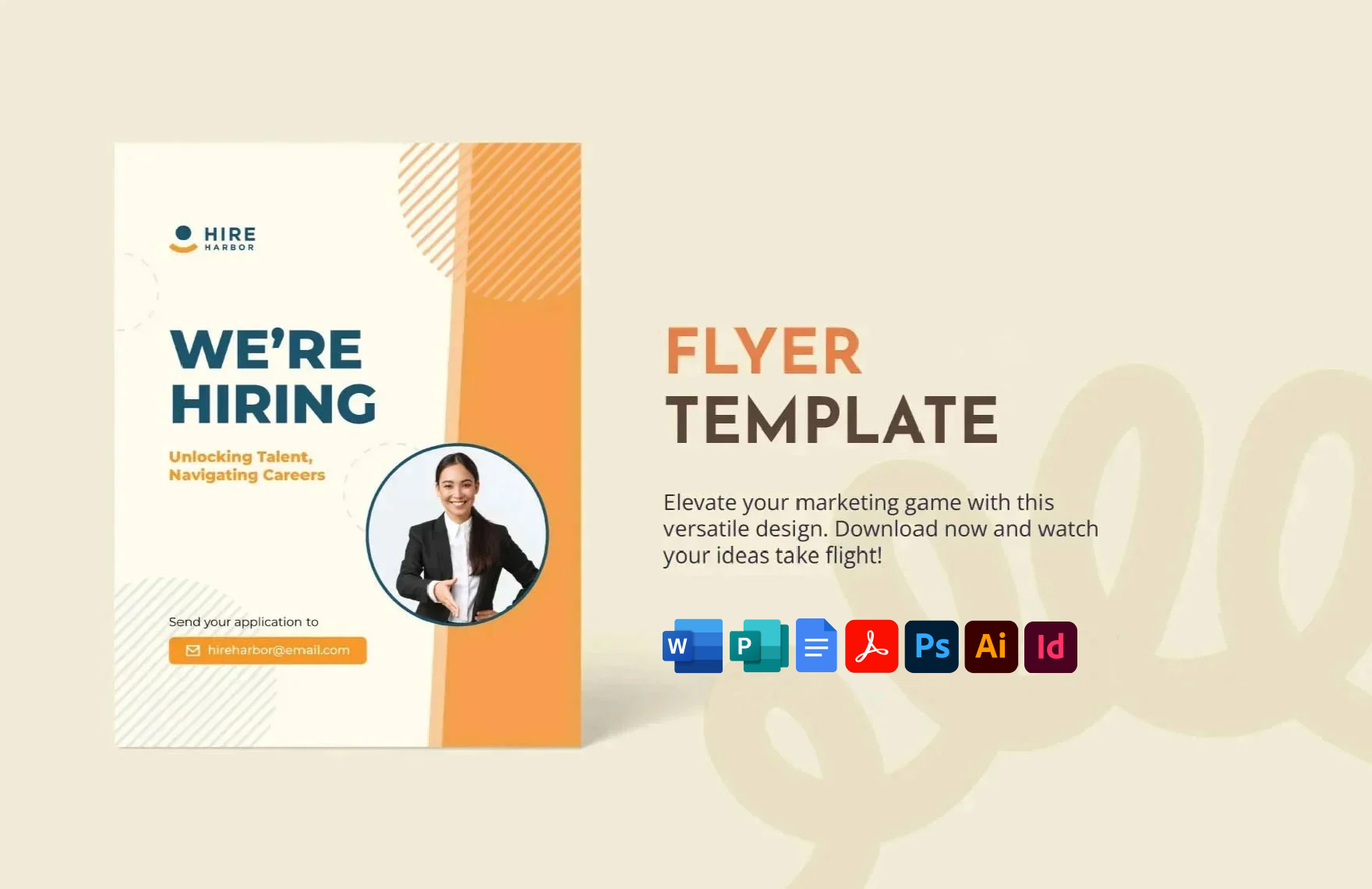The image depicts a professionally designed, horizontal business card or website page aimed at marketing and design. It's set on an ivory background and primarily features an advertisement for a hiring flyer template by Hire Harbor. Dominating the left side of the image, bold green and blue letters announce "We're Hiring," followed by the tagline "Unlocking Talent and Navigating Careers" in yellow and tan. A professionally dressed woman in a white shirt and dark blazer, smiling with her hand extended for a handshake, is prominently displayed within a circle. 

To the right, an advert for the flyer template is showcased with the words "FLYER TEMPLATE" in orange and brown letters respectively. Below that, gray text reads, "Elevate Your Marketing Game with this Versatile Design. Download Now and Watch Your Ideas Take Flight." Symbols indicating compatibility with various design programs like Word, Publisher, Docs, Adobe Reader, and Photoshop are lined up underneath. The bottom right corner features faint yellow squiggly lines reminiscent of a telephone cord, enhancing the creative layout. The color scheme harmonizes brown, white, green, yellow, orange, blue, black, and red, giving a balanced and visually appealing look.